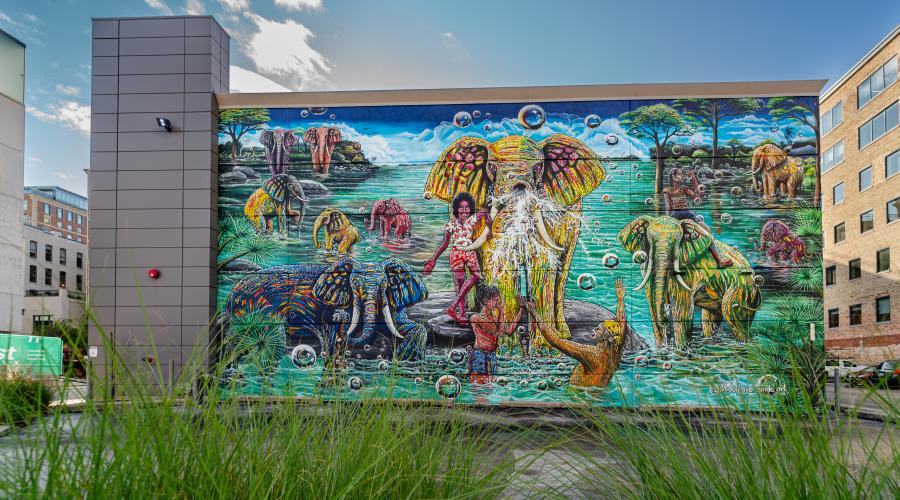In the image, there is a large, flat-roofed building adorned with an intricate mural depicting a vibrant, surreal scene of elephants bathing in a water area. The mural showcases a variety of elephants painted in bright, vivid colors such as yellow, blue, green, red, and purple. The central figure is a predominantly yellow elephant gazing towards the camera with a mix of pink, blue, and orange hues. On the left, a blue elephant rests on a rock, while on the right, a green elephant stands upright, also facing the camera. Additional colorful elephants can be seen in the background, including red and yellow ones. Some of the elephants appear to be interacting with people, as three shirtless men in shorts are depicted splashing water and helping the elephants bathe, with one person even hanging off the main elephant's trunk.

In the surroundings, a blue sky forms the backdrop with buildings to the left and right of the mural. To the right, a brown building with multiple windows, suggestive of a hospital or office, stands tall. In front of the mural, a parking lot with several parked cars is visible, partially obscured by tall green grass. The left edge of the mural building has no windows and features a security light and an alarm system, adding to the industrial feel against the otherwise bright and whimsical mural.